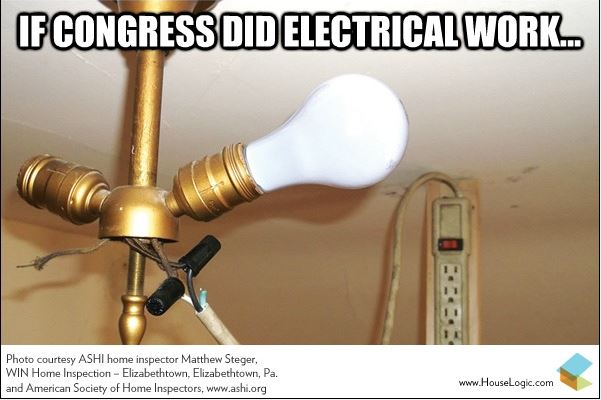The image is a horizontally aligned rectangular meme with a black border on the sides and bottom. At the top, there is a large white, all-caps text with a black outline that reads, "IF CONGRESS DID ELECTRICAL WORK..." The focal point is a light fixture hanging from the ceiling, colored bronze or gold. The fixture has two light sockets, one on the right with a light bulb inserted, and one on the left without a bulb. Beneath the fixture, multiple exposed wires are visible, indicating very shoddy and unsafe electrical work. The wires on the right are linked together with a wire nut, while the wire on the left is uncapped and exposed. The image shows the wiring leading to a power strip mounted on a piece of plywood attached to the wall. The bottom part of the picture has a white background with text that says, "Photo courtesy ASHI, Home Inspector Matthew Steger, When Home Inspection-Elizabethtown, Elizabethtown, PA, and American Society of Home Inspectors www.ashi.org" on the left, and "www.houselogic.com" on the lower right-hand corner. The overall scene appears dingy and poorly executed, enhancing the meme's satirical take on Congress's competence.